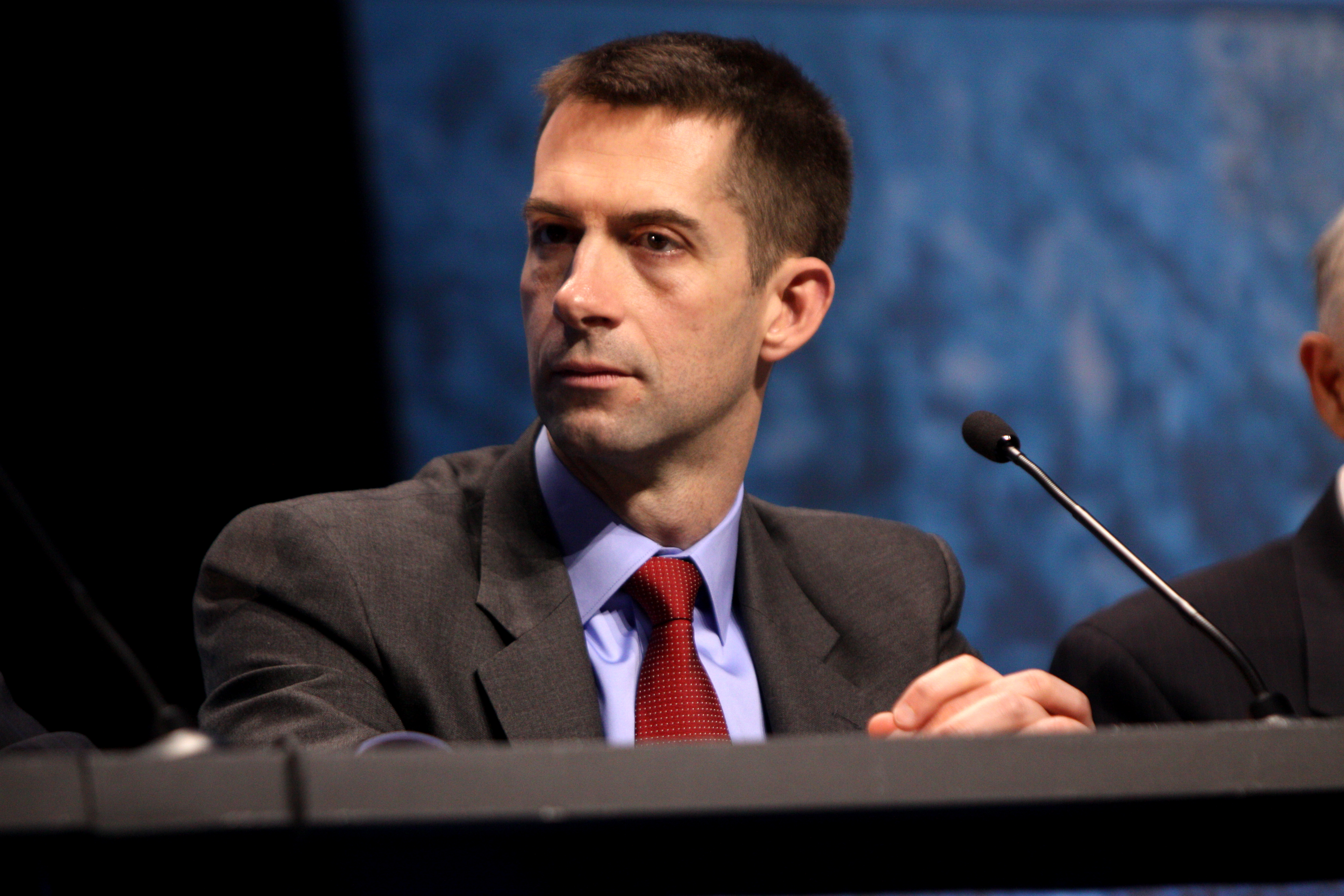The image depicts a close-up of a middle-aged man seated at a podium, likely part of a panel discussion or press conference. The man has short brown hair, described variously as cut fairly short or like a crew cut, and brown eyes. His facial expression is neutral, suggesting he is deep in thought as he gazes to his right. He wears a dark grey suit with a light blue button-down shirt and a red tie tied in a Windsor knot. He has his hands folded in front of him above the table, and a thin black microphone with a fuzzy black tip is positioned in front of him.

In the background, there is a mixture of blue and black walls, adding depth to the setting. To the left of the main subject, you can partially see another man, identifiable only by his shoulder, the side of his head, and some gray hair. The overall scene conveys a formal, professional atmosphere, with the main subject seemingly engaged or preparing to engage in a discussion or presentation.